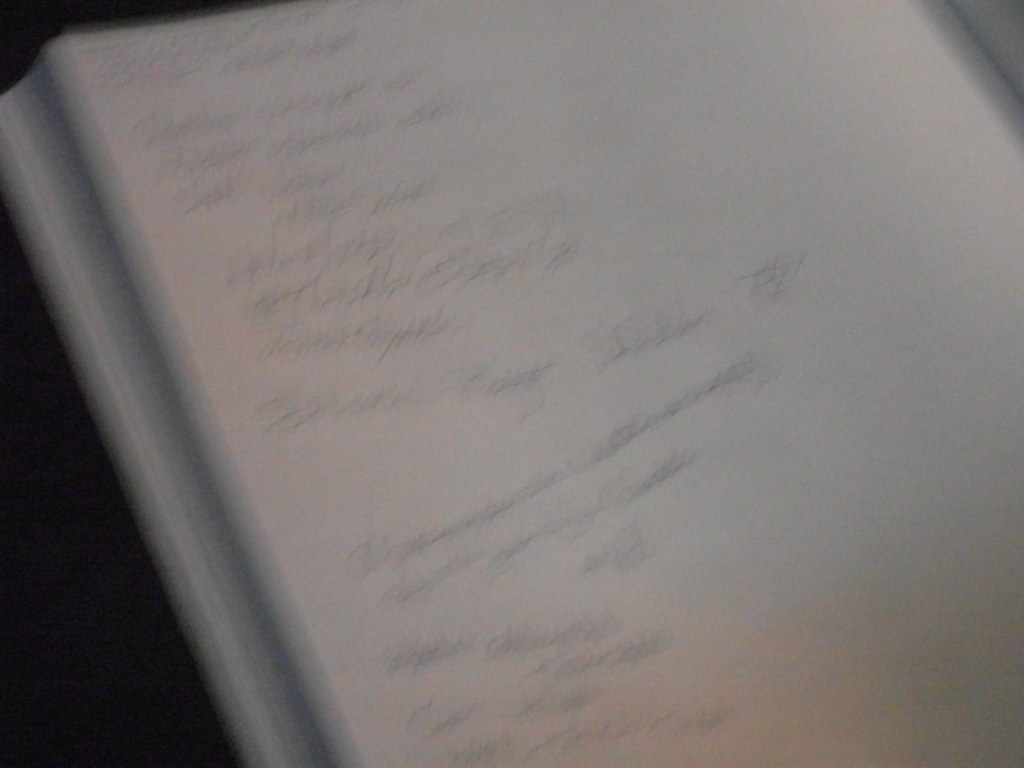The image is a very blurry, low-quality close-up photograph likely taken in low lighting, which results in a predominantly black and white appearance. It features an open page inside a book, with a noticeable emphasis on the left side of the page where most of the writing is concentrated. The text appears to be written in either pencil or pen, with some sections in fine print being illegible due to the blurry nature of the photo. There are various orientations of the scribbles, with some words written sideways or even crossed out, giving the impression of a sketch or notes taken in a haphazard manner. The surface of the page is white, contrasting against a solid black background seen behind the book. The top left corner of the sketchbook is visible, while the right side of the page appears mostly empty, almost resembling a list format. The bottom of the image shows darker scribbles, possibly smudged by an eraser.